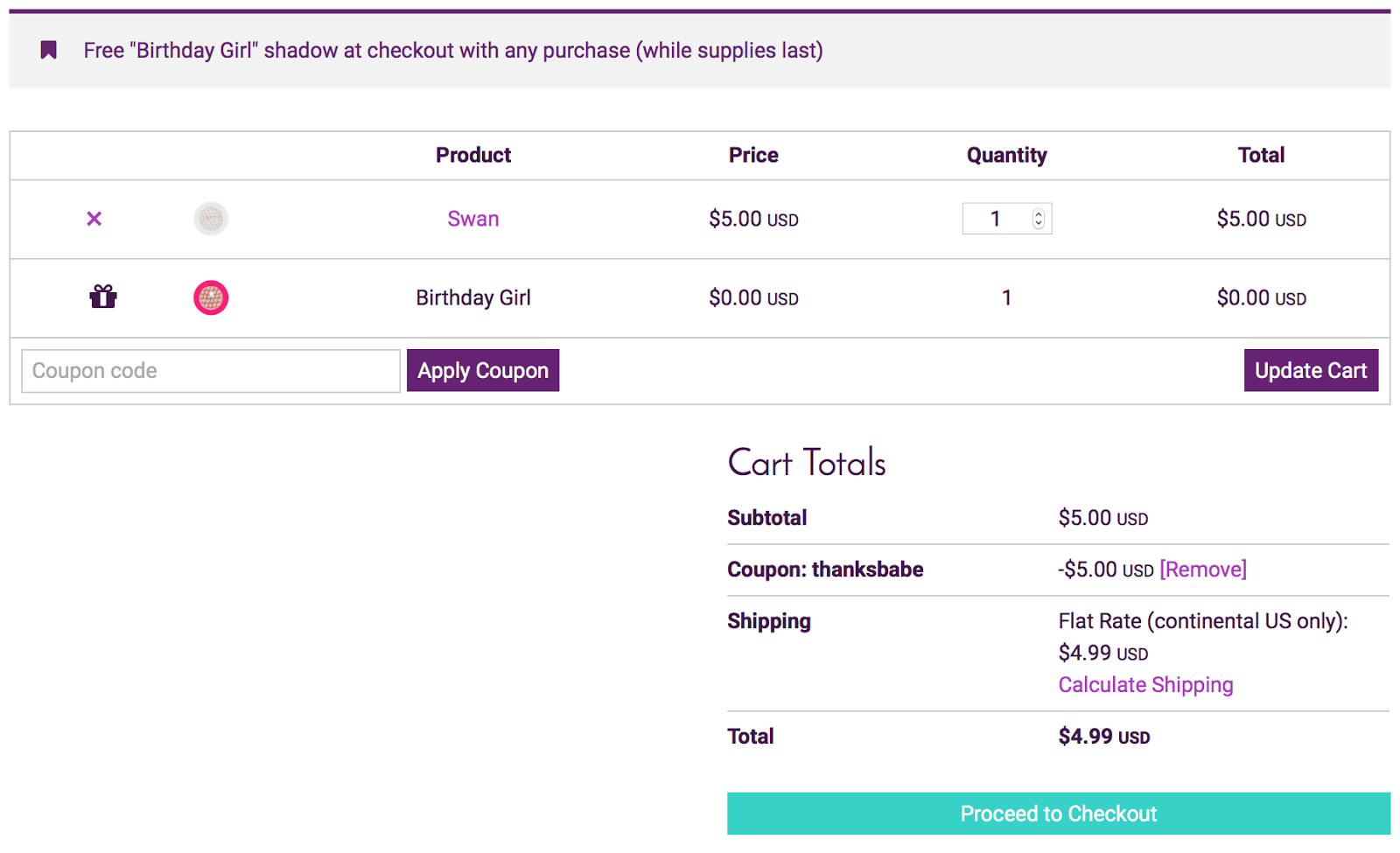Screenshot Description: 

This screenshot showcases the cart page of a website, characterized by a light creamy purple background and dark purple text. At the top of the page, a promotional banner highlights a special offer: "You get a free Birthday Gift at checkout with any purchase while supplies last."

Below the banner, the cart displays two products. The first product, named "Swan," is listed at a price of $5.00, while the second product, "Birthday Girl," is listed at $0.00, indicating that it was received as a free gift in accordance with the promotional offer. Each product has a quantity of one.

Further down, there is an option to enter and apply a coupon code, indicated by a purple button. In the bottom right corner of the page, the cart totals are presented, showing a final amount of $4.99 USD.